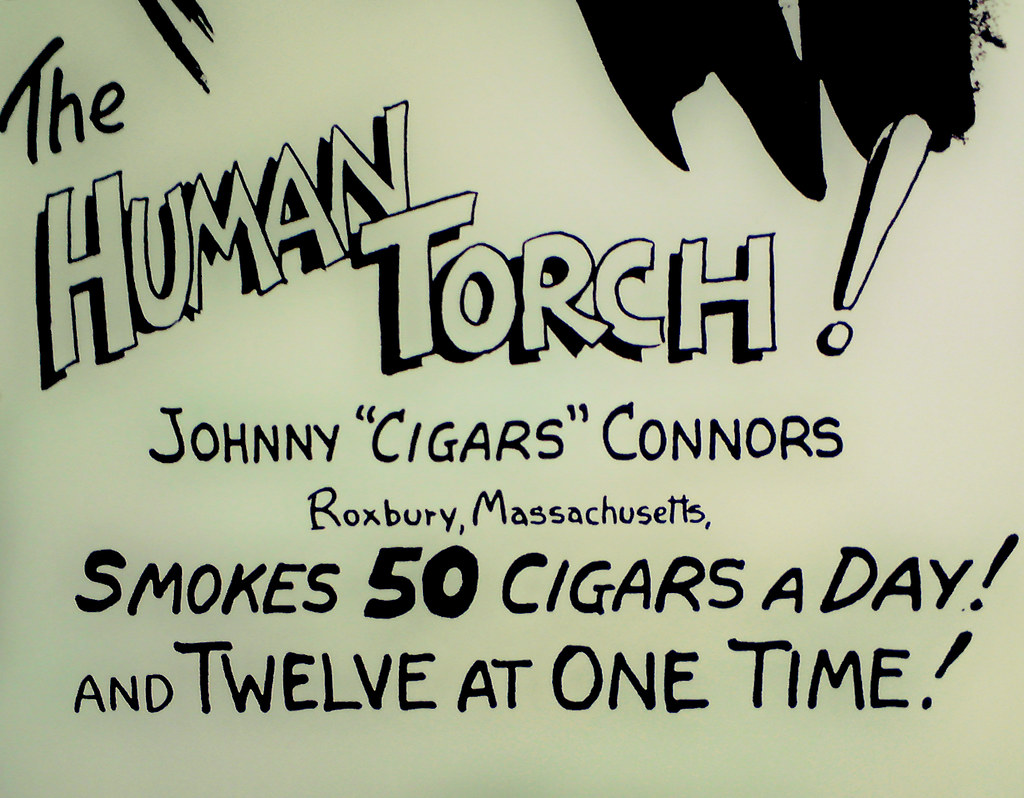The image features bold black text on a light blue background. The upper left corner has the words "This is where the words start," with the text cascading downward. The headline reads "The Human Torch! Johnny 'Cigars' Connors, Roxbury, Massachusetts, smokes 50 cigars a day, and 12 at one time!" The text "Human Torch!" is written in bubble letters with an exclamation mark, while the rest of the text is in a dark, shadowy font. In the upper right corner, there are two thick black streaks of paint, and two smaller black markings are visible in the upper left corner, though their purpose is unclear. The background is predominantly a light blue or light green military shade, with no images of people or objects, making it a simple yet intriguing promotional ad likely aimed at drawing attention to Johnny 'Cigars' Connors and his unique cigar-smoking prowess.